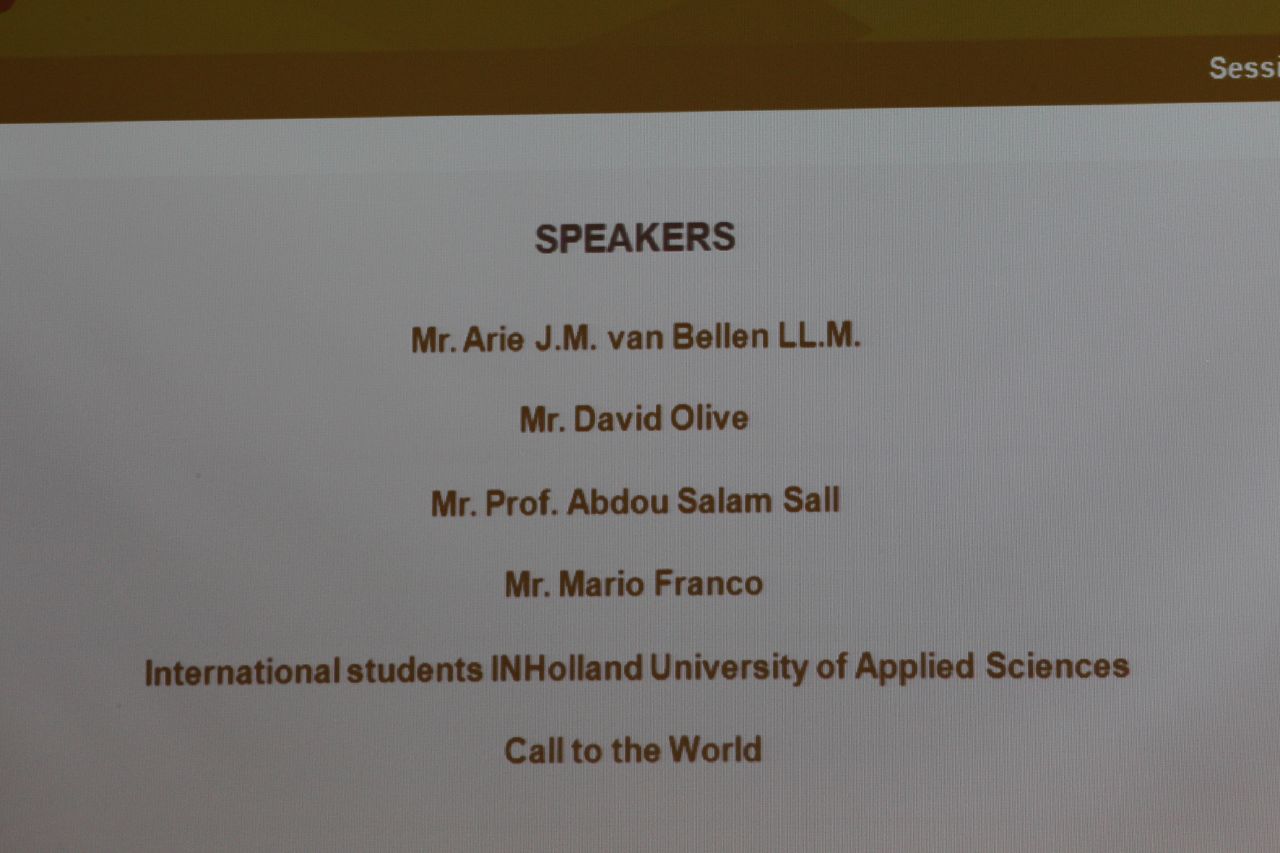The image depicts an off-white card with a white background featuring a list of speakers for a conference or seminar. At the top, in bold black letters, it says "Speakers." The speakers are listed below in brown lettering. From top to bottom, they include:

1. Mr. Arie J.M. Van Bellen, LL.M.
2. Mr. David Olive
3. Professor Abdo Salam Sall
4. Mr. Mario Franco

Following the individual speakers, the card lists "International Students in Holland, University of Applied Sciences" and ends with "Call to the World." The image, which appears pixelated like a photograph of a projected slide or computer screen, provides a clear overview of the event’s scheduled speakers.